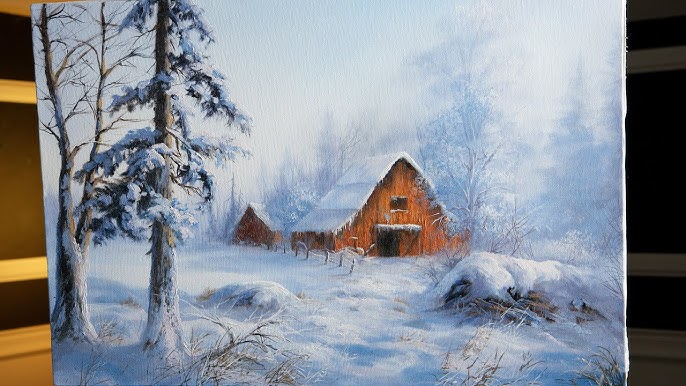The image is a photograph of a painting that depicts a serene winter scene, evocative of a Bob Ross landscape. The painting captures an outdoor setting on what appears to be a canvas. In the foreground, on the left side, stand two tall trees—a snow-covered evergreen and a leafless tree with bare branches. A field stretches out from the front, dotted with brown vegetation poking through a thick layer of snow. Just behind the trees, there's a rustic barn with a white, snow-covered roof. The barn's brown, perhaps yellowish, wooden exterior adds a touch of warmth amidst the cold scenery. Adjacent to the barn, another smaller building or house is somewhat visible, continuing the snowy theme. Further back, a line of shadowy, snow-covered trees fades into a foggy background, creating a depth-enhancing, almost ethereal atmosphere. The photograph displaying the painting is taken indoors, with a well-lit wooden shelf visible to the left and an empty, shadowy shelf on the right, adding context and contrast to the displayed artwork.